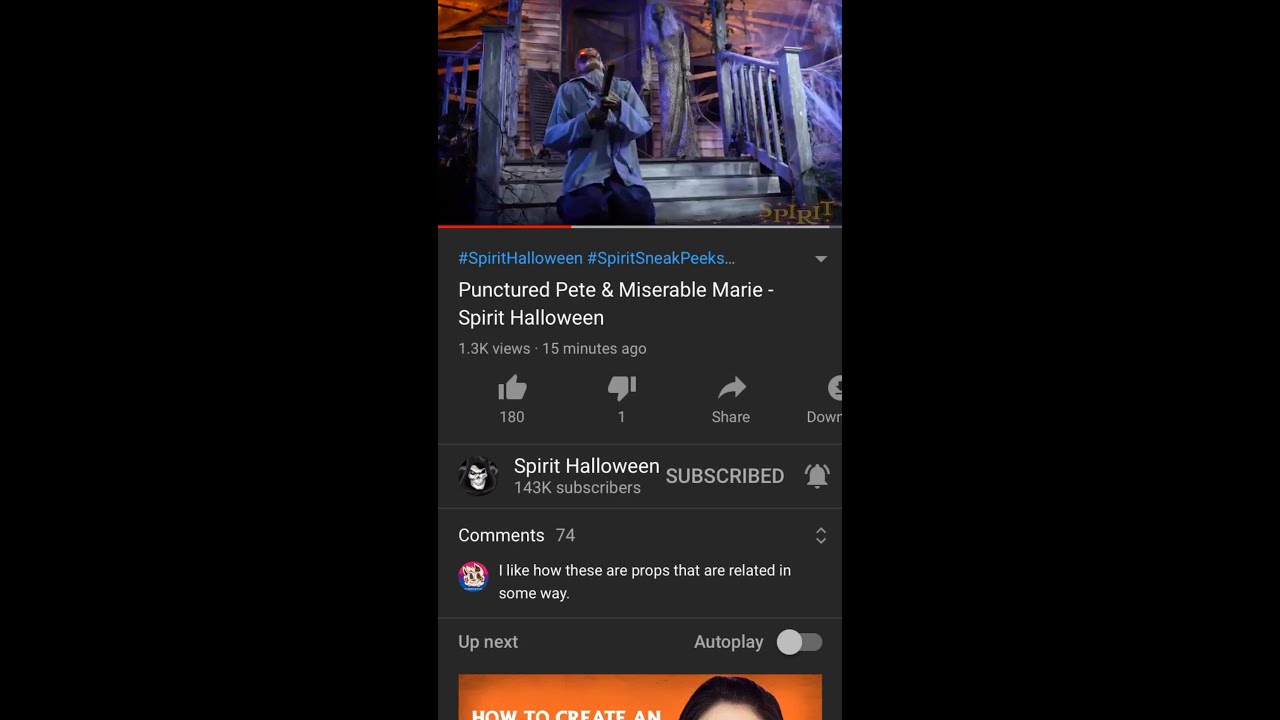The image features a YouTube video playing in the center with a solid black background on both sides. At the bottom of the video, an orange rectangle is partially visible. On the right side of this rectangle, there is an individual’s forehead with brown hair. The title of the video reads "How to Create Anne," although the bottom part of each letter is cut off. Above the video title, the text "Up Next" is displayed in white. 

To the right, the words "Order Play" (most likely part of the "Autoplay" function) are visible, underlined by a thin white and gray line. A comment is displayed beneath the video, with a user profile image resembling a doll against a pink, purple, and blue background. The comment text, in white, reads: "I like how these are props that are related in some way," and is marked as comment number 74.

Above the comment, the YouTube channel name and details are present. The channel's profile image is a black Grim Reaper icon next to the name "Spirit Halloween" with capitalized initials. The channel has 143K subscribers, and buttons for subscribing and the notification bell are present. 

The video has received 180 thumbs up, one thumbs down, and buttons for sharing and downloading (partially cut off) are shown. The video has 1.3K views and was posted 15 minutes ago. The video title reads "Puncture Pete and Miserable Mary Spirit Halloween," followed by the hashtags #SpiritHalloween and #SpiritSneakPeeks in blue text. The video thumbnail appears to show a fake character lying on a stair.